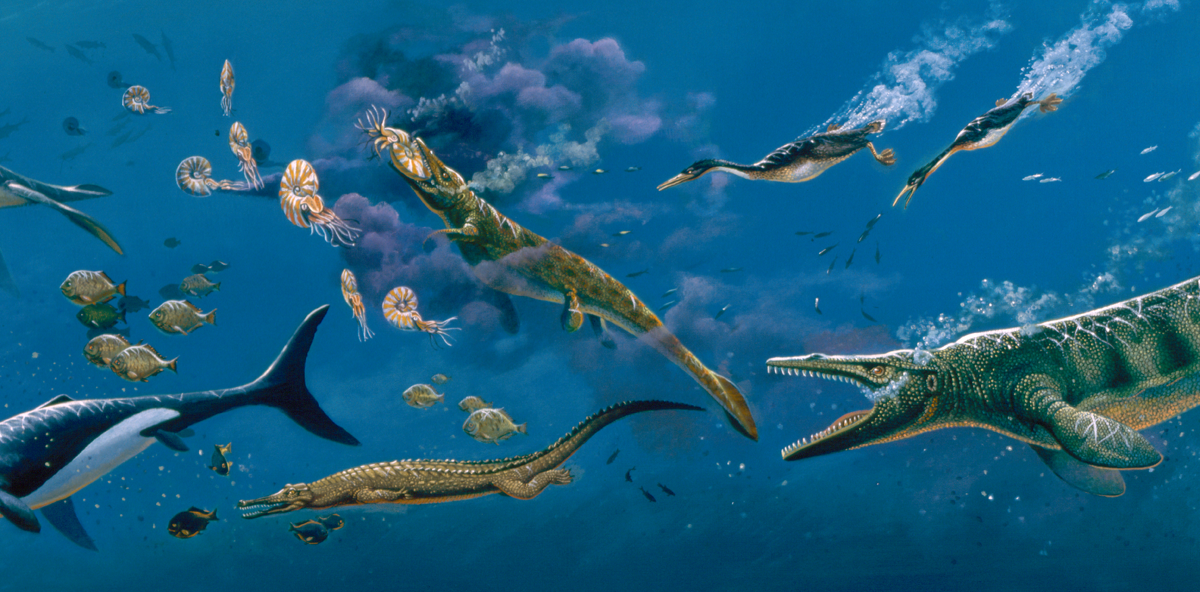This captivating digital illustration features a surreal underwater scene teeming with fantastical creatures. Dominating the bottom right of the image is a unique hybrid resembling a cross between a crocodile and a manatee. This creature boasts a lizard-like head with its mouth wide open, revealing several rows of small, spiky teeth. Its body is equipped with fins akin to those on a manatee or a sizable fish, enhancing its mythical appearance.

Adding to the intricate detail, several black waterfowl, reminiscent of geese but with diving tendencies, are shown plunging into the water in pursuit of fish. These birds display striking white bellies and vivid yellow beaks. Another of the crocodile-manatee hybrids can be seen deeper within the scene, feasting on a peculiar, giant, snail-like creature adorned with tentacles.

The bottom left corner of the illustration reveals a portion of a killer whale's tail, just below a creature that resembles a crocodile even more closely. This second crocodilian entity maintains the characteristic shape, legs, feet, and tail of a crocodile, but its head is distinctly pointier.

Scattered throughout the scene are various fish swimming amidst a backdrop of deep blue hues. Bubbles ascend gracefully from the mouths of the creatures, contributing to the dynamic underwater atmosphere. Enhancing the sense of enchantment, a smoky, cloud-like effect drifts upwards from the ocean floor, suggesting the aftermath of an underwater explosion and adding a dreamlike quality to the entire composition.